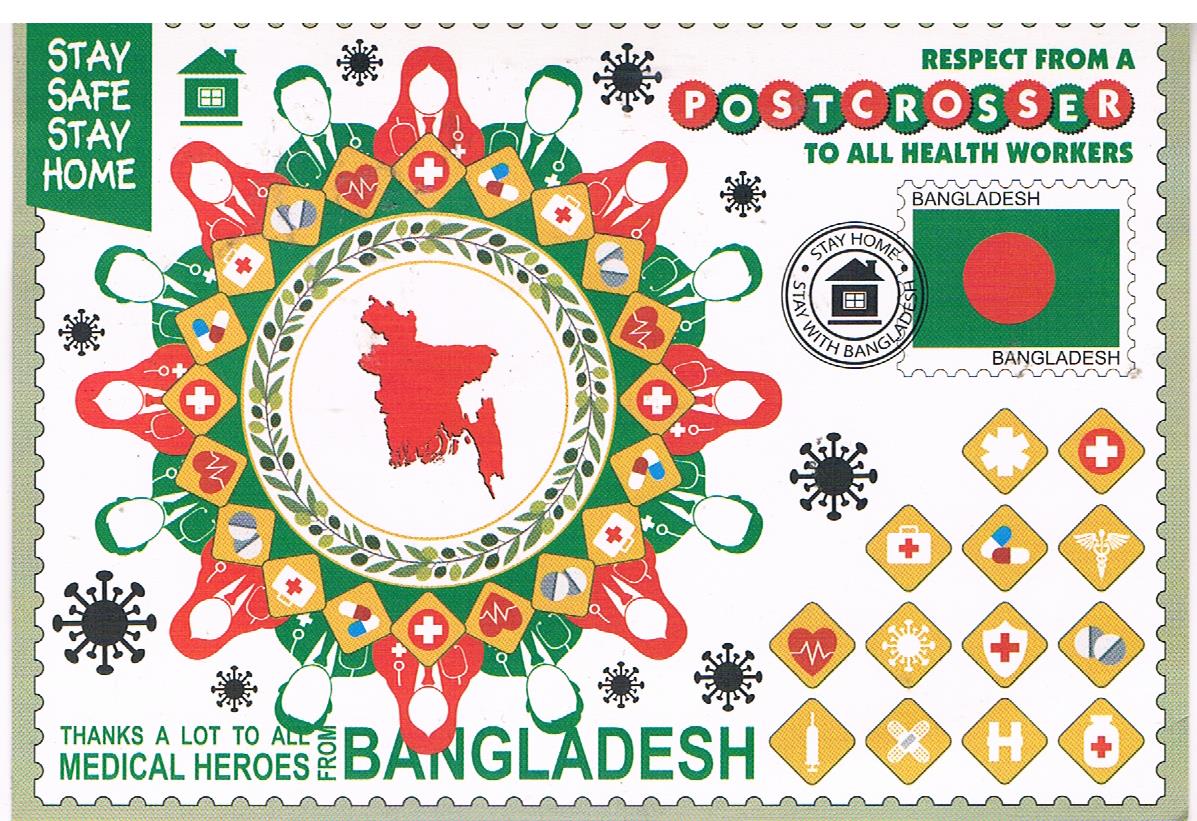The image features a detailed and symbolic postcard dedicated to honoring healthcare workers during the COVID-19 pandemic in Bangladesh. The postcard's background resembles a green mesh canvas, while its main section, designed to mimic a postage stamp with a white backdrop and perforated edges, showcases a central map of Bangladesh surrounded by faceless illustrations of doctors and nurses. The predominant colors used are green and red.

In the upper right-hand corner, a heartfelt message reads, "Respect from a post crosser to all healthcare workers." Below this, a red circular stamp framed by a green square bears the word "Bangladesh." Nearby, another stamp urges, "Stay home, stay with Bangladesh." The upper left-hand corner displays the words, "Stay safe, stay home," reinforcing the pandemic context.

Scattered around the postcard are various medical icons, including a cross, medication, an emergency kit, a heart with a pulse line, and other healthcare-related symbols. The images also include black outlines representing the COVID-19 virus, further emphasizing the period during which this postcard was created.

At the bottom, a touching message extends gratitude, saying, "Thanks a lot to all medical heroes from Bangladesh." These collective elements come together to convey a deep appreciation for the tremendous efforts of healthcare workers during the global health crisis.